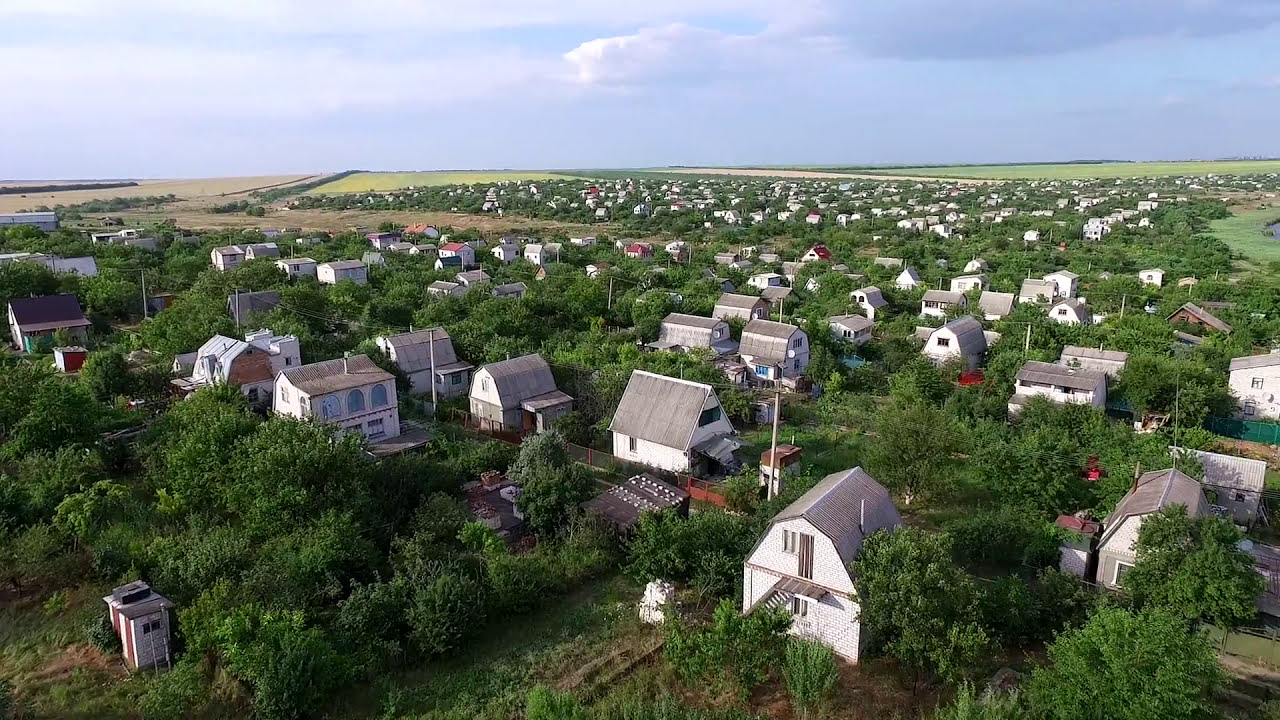This photograph, seemingly taken from an elevated vantage point, possibly by a drone, showcases a quaint town spread across a large, flat area. The town features numerous two-story houses, each characterized by their white exteriors and uniform gray, triangular-shaped roofs. These homes are spaced widely apart, with ample gaps between them filled by a lush expanse of greenery. Trees are abundant, surrounding and interspersed among the residences, creating a serene, natural environment. The horizon line occupies the upper 20% of the image, marking the transition between the town and a vast expanse of sky. The sky is predominantly blue, dotted with a few clouds, adding to the picturesque and tranquil setting of this seemingly close-knit community.